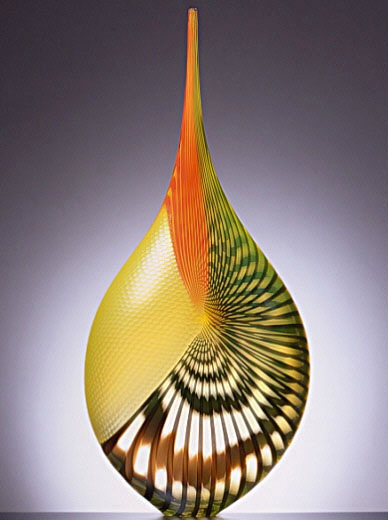This is a detailed depiction of a tall, rectangular artwork with a gradient background that transitions from a darker light grayish purple at the top to a lighter shade towards the bottom. Situated prominently in the center of the image is a glass-designed object resembling a teardrop. The shape is broad at the bottom and narrows to a pointed peak at the top. The left side of the teardrop features a shiny yellow and orange scaly surface with orange stripes extending upwards. Adjacent to this, the object's bottom right side transitions into a striped pattern with dark green stripes and green horizontal circles on a light yellow background, reminiscent of a seashell design. Further up, the object exhibits brown and white striated patterns, akin to the intricate designs found on monarch butterfly wings. The teardrop-shaped object appears illuminated by a light source from the rear center, adding depth and dimension to its shiny, textured surfaces.